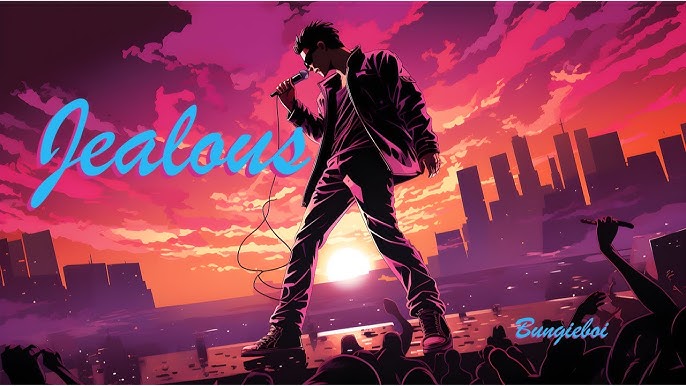The image depicts a stylized cartoon poster featuring a male singer standing on a stage, holding a microphone with a long cord. He has short, spiky, slicked-back hair and is wearing dark sunglasses. His outfit consists of a relatively close-fitting, yet wrinkly-looking black ensemble, including a dark jacket, shirt, pants, and black sneakers with white laces. He stands with his legs apart, singing passionately to a large crowd beneath him, whose figures are darkened by shadows.

The vibrant background showcases a stunning sunset with an array of colors including orange, yellow, pink, and purple, blending into a darkening sky. The sunset is visible between the singer's legs, enhancing the dramatic effect. Behind him is a city skyline of tall, purplish-gray skyscrapers, adding depth to the scene. Prominently featured in light blue cursive font is the word "Jealous," positioned next to the singer. In the bottom right corner, the name "Bungie Boy" is displayed, stylized as "B-U-N-G-I-E B-O-I."